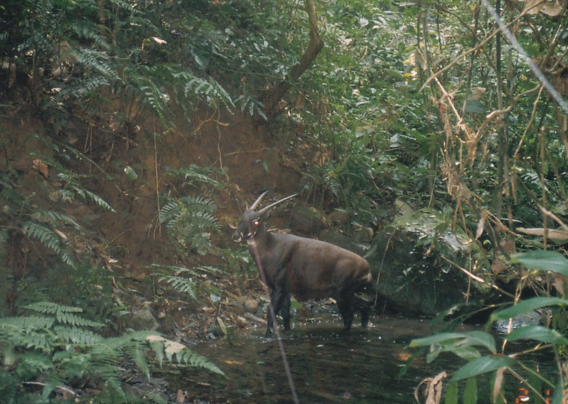In this color landscape photograph, set within a dense, lush forest, stands a Saola, an elusive and rare horned creature often mistaken for a deer. This vibrant image captures the Saola in profile, positioned near the center bottom of the frame, its head facing left. The animal boasts a dark brown coat with distinct white markings on its nose and neck, accentuating its unique appearance. Two long, straight beige horns extend backward from the top of its head. The Saola's short black legs are partially submerged in an ankle-high pond of water, adding a reflective element to the scene.

The environment around the Saola is richly vegetated, with various green plants, including ferns and traditional leaves, some fresh and others dried up. The dense foliage is so thick that it obscures the sky, creating an encapsulated jungle atmosphere. In the background, a sizable hill covered in trees and grass rises, further enhancing the forest feel. Despite a small stick partially obstructing the face area of the Saola, the creature's glowing eyes, likely a result of camera flash, are visible and add an intriguing detail to the photograph. This image exemplifies photographic representationalism realism, capturing the Saola and its natural habitat in intricate detail.